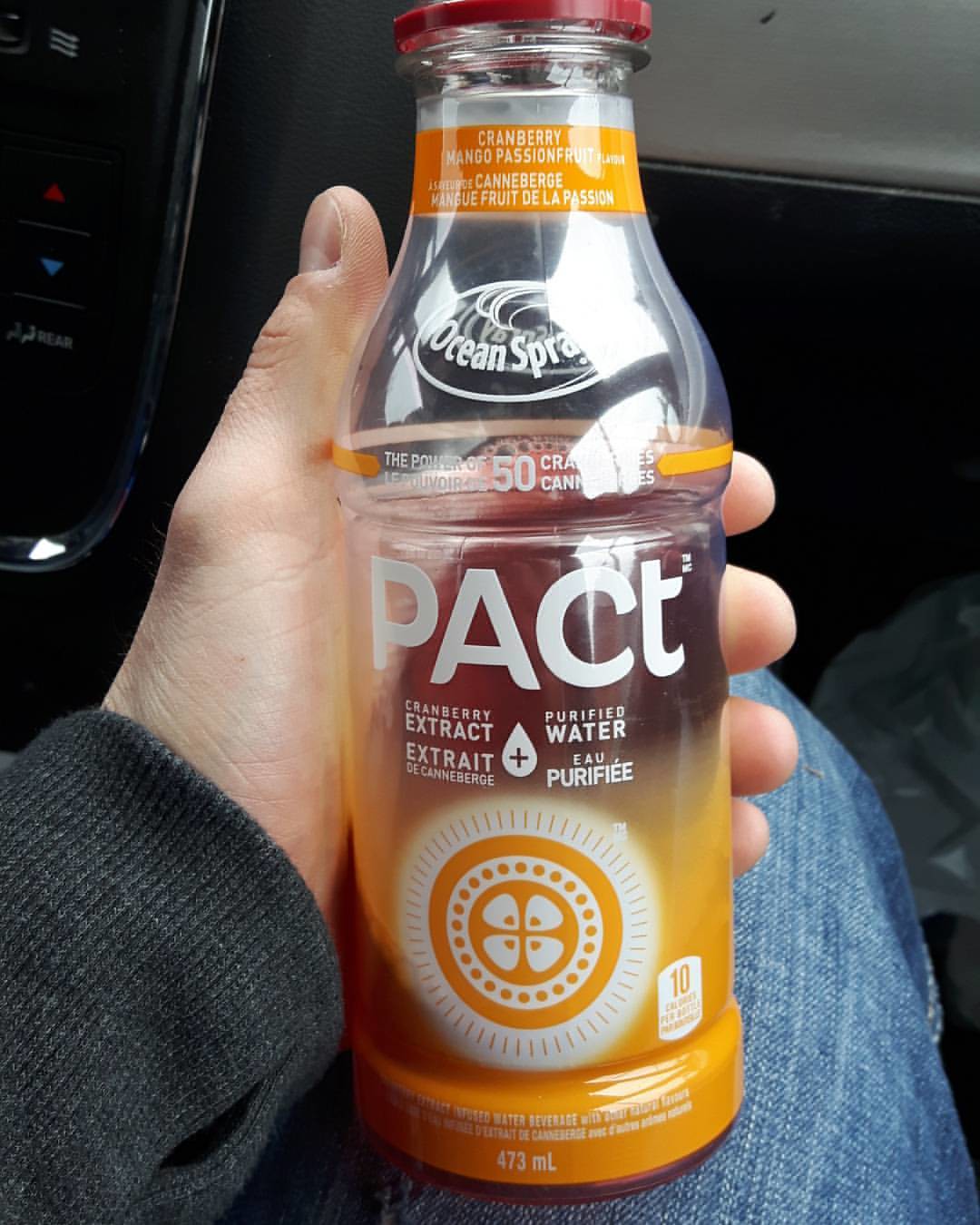This image captures a close-up of a Caucasian man sitting in a car, holding a clear, likely plastic bottle with distinct orange and red branding. The man, dressed in a grayish-black sweater and blue jeans, has the bottle nestled in his left hand, prominently displayed at the center of the photograph. The bottle, identified as Ocean Spray's PACT, features cranberry extract in purified water. The branding includes a mix of white and orange accents, with 'PACT' inscribed in large white letters on the front. 

The bottleneck is adorned with an orange tab and the Ocean Spray logo, which includes a small wave design. Below it, the yellow band wrapping partially around the bottle contains some product information, though it’s partly obscured by the lighting. More noteworthy details include the product's volume of 473 milliliters and phrases like 'the power of flavor' and '10 calories,' with the latter confirmed in both English and French.

The intricate design at the bottle's bottom features a white medallion with a four-leaf clover in the center, circled by various radial markings. Despite the slight blurriness in parts, the overall presentation is clear, emphasizing the man's grip and the detailed labeling of the bottle. In the background, one can glimpse the car's interior, including part of a cell phone in the upper left corner, adding context to the setting.